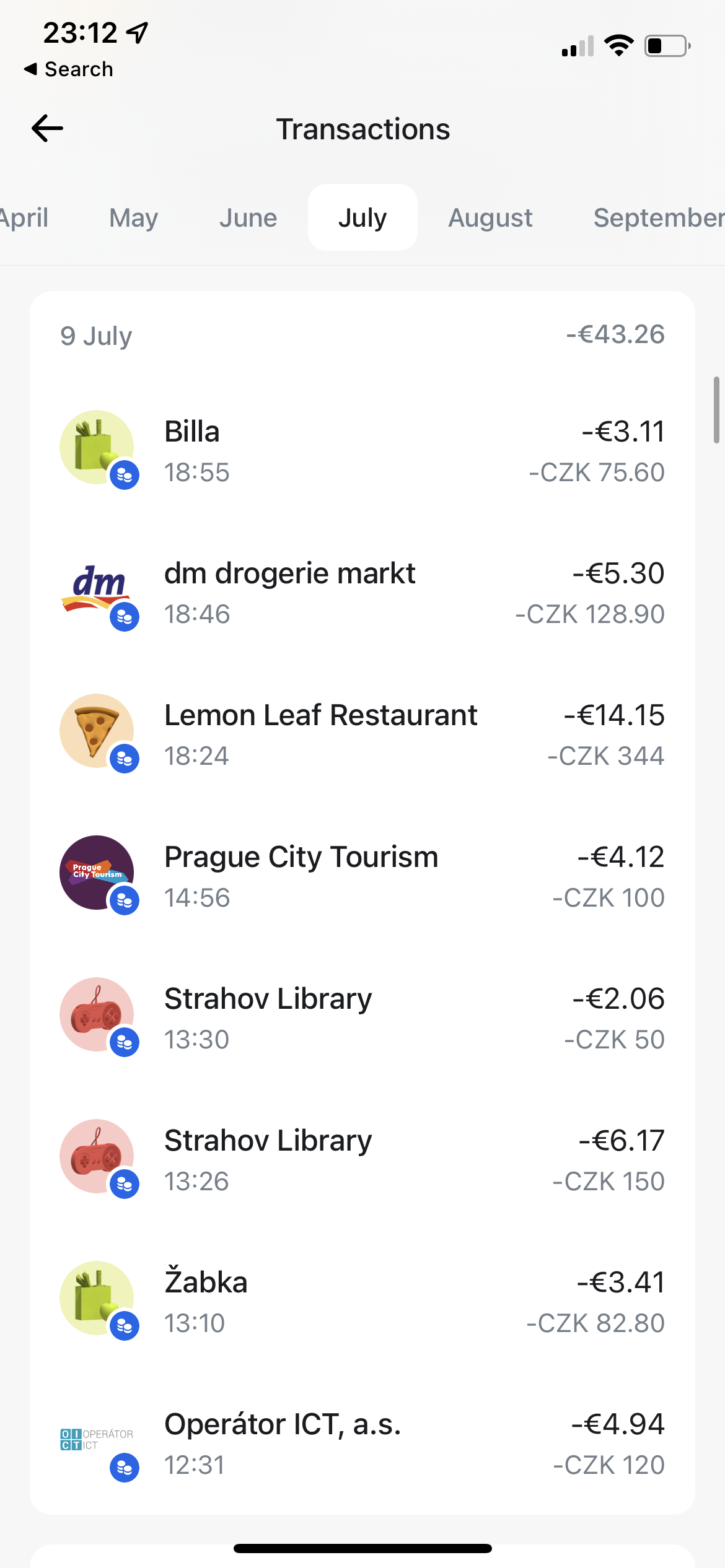A detailed screenshot display from a mobile banking application showcases various elements and transactions. 

**Top Section:**
- **Time and Status Indicators:**
  - At the very top left, the time reads "23:12."
  - Adjacent to the time, battery percentage and mobile service signal icons are visible.
  
**Search and Navigation:**
- Below the status bar, a small black text box reads "Search," accompanied by a left-pointing arrow.
- Another larger left-pointing arrow is situated below the search bar.

**Transaction Header:**
- Directly below the navigation arrows, the word "Transactions" is presented in black text.

**Date Selection:**
- The range of months displayed spans from April to September, albeit partially cut off at the ends.
- The month of July is highlighted, indicating it's the selected period.

**Transaction List for July 9th:**
- A series of transactions is listed for July 9th (or the 9th of July). Here are the entries along with their details:
  1. **Billa:** $43.26
  2. **DMTROGRIE Markt** (market spelled as "MARKT")
  3. **Lemon Leaf Restaurant**
  4. **Prague City Tourism**
  5. **Strahov Library**
  6. **Zabka**
  7. **Operator ICTA.S.**

Each listed transaction option accompanied by respective prices, though only the first transaction (\$43.26 at Billa) has the amount specified in the description.